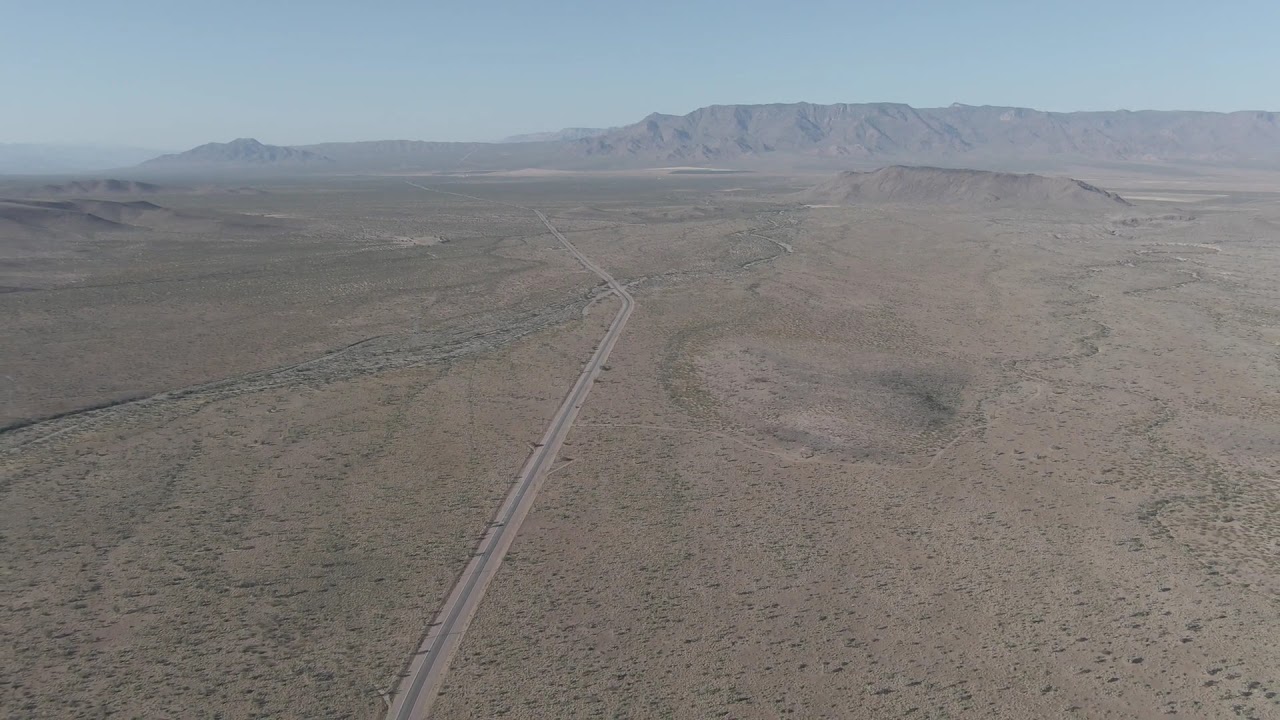The image is a large, panoramic aerial view of a desolate, dry desert landscape dominated by a long and winding highway that stretches through the center. The ground is predominantly brown, broken up by patches of green sagebrush and small trees. Notably, the desert surface features various mounds of dirt, hills, and a prominent crater on the right-hand side of the road, with dark shadows indicating its depth. There’s also a hollowed-out area that may have once been a pond, situated centrally amid open fields on the left of the road. In the background, an extensive range of rocky mountains spans the horizon beneath a hazy, blue sky, creating a striking contrast to the barren foreground.